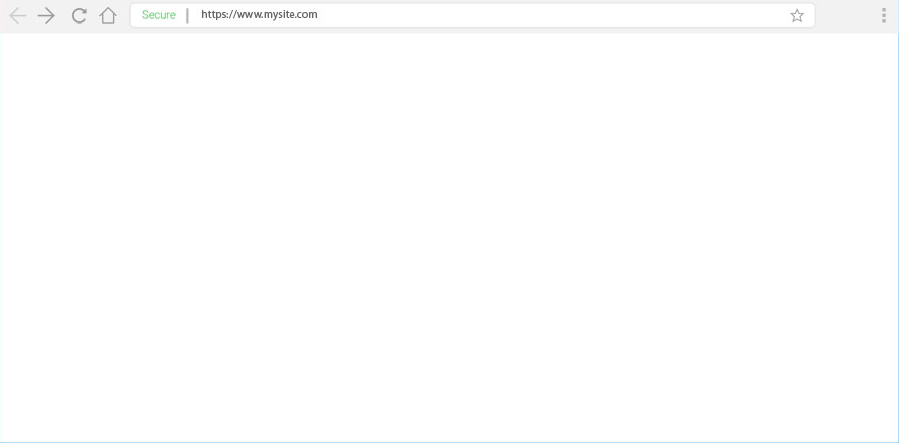The image depicts a web browser window with a minimalistic interface. At the top of the window is a small gray bar that houses a search bar, where the URL "https://www.mysite.com" is displayed. To the left of the URL is a green padlock icon, indicating that the site is secure. The search bar also includes standard browser features such as a star icon for bookmarking the page and arrows for navigating forward or back to different pages. However, the main content area of the browser window is entirely blank, suggesting that the Enter key has not been pressed or that the website has not loaded any content. The absence of any visual or textual information on the page emphasizes its stark emptiness.